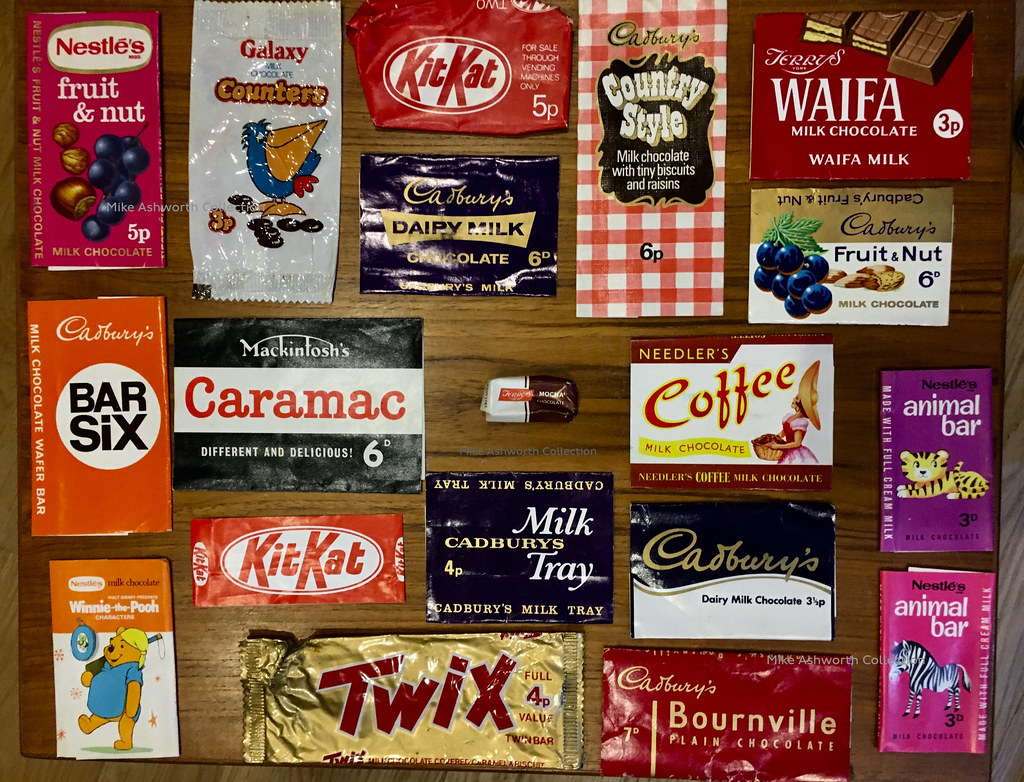The image is a detailed photograph taken from a top angle, depicting a variety of chocolate and candy bars spread out on a wooden brown table. The collection, arranged in rows and columns though not very neatly, features both modern and vintage wrappers. Brands such as Nestle, Cadbury, and Macintosh are prominently displayed. In the top left corner, you can spot Nestle's offerings, including Fruit and Nut and assorted Animal Bars with tiger and zebra illustrations. The bottom right corner shows various Cadbury chocolates such as Dairy Milk, Barnville Plain Chocolate, Milk Tray, and fruity options with tiny biscuits and raisins. There’s also the vintage Needler's Coffee Chocolate with a distinctive wrapper featuring a woman in a pink dress and sombrero-type hat. Additionally, Twix and multiple KitKats can be seen scattered around the table. Some wrappers, like Galaxy Counters and Macintosh Caramac, hint at the age of some products with their retro designs. A watermark reading "Mike Ashworth collections" is visible on the image, suggesting the curated nature of this display.